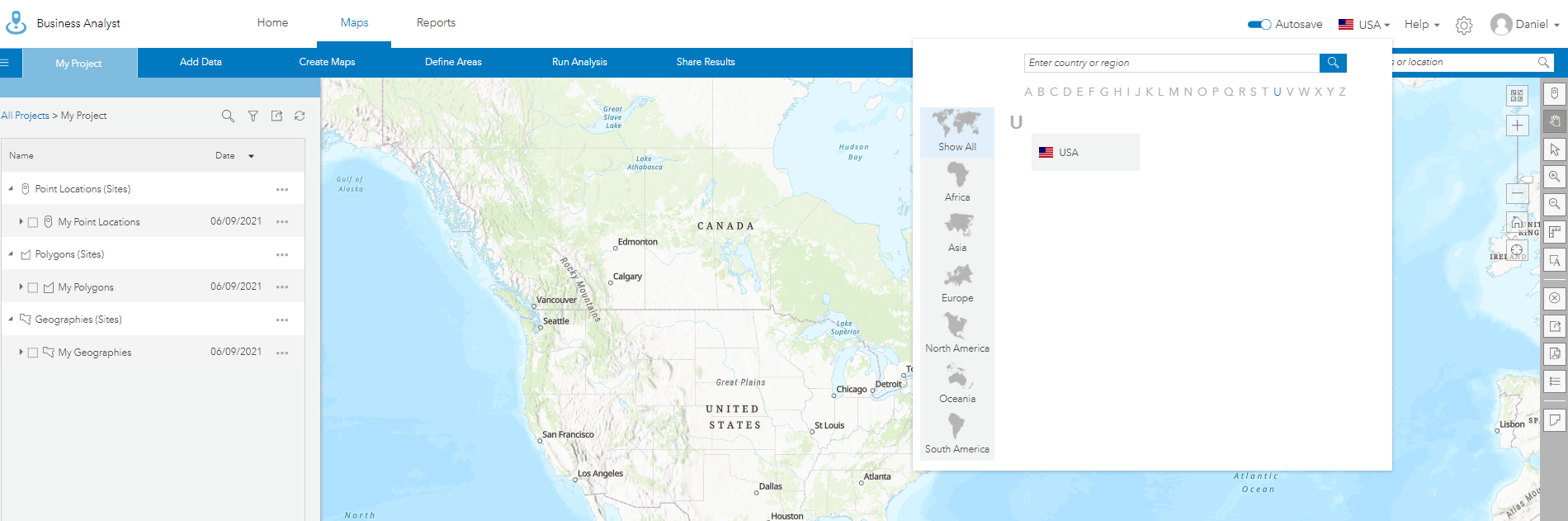Desktop application screenshot displaying the interface of a Business Analyst tool. Positioned at the top left is the title, "Business Analyst". Adjacent to this title are multiple navigational tabs. The "Maps" tab, centrally located, is active, flanked by the "Home" tab to its left and the "Reports" tab to its right. On the far-right side of the navigation bar is the "Auto Save" toggle, currently enabled. Further right, there's a "Country" dropdown menu set to "USA", followed by a "Help" dropdown, and a gear icon signifying settings. The user's profile, labeled "Daniel" without a profile photo, is positioned at the extreme right, also with a dropdown menu.

Directly below the Auto Save toggle and the USA dropdown is a search input field adorned with a magnifying glass icon, denoting functionality for searching countries or regions. Below this search field, alphabetical tabs labeled A to Z are visible, with the letter "U" currently selected, indicating "USA". To the left of the alphabetical navigation are two options, where "Show All" is chosen. Below these, continent options are listed: Africa, Asia, Europe, North America, Oceania, and South America.

The main screen presents an enlarged world map prominently focused on Canada and the United States, providing a geographical context to the selected options.